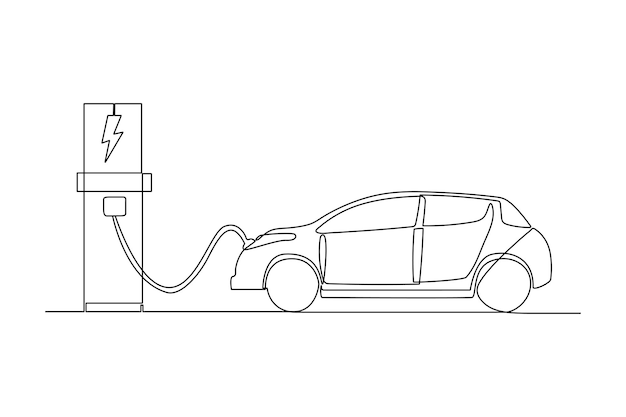The image is a highly simple black-and-white line drawing depicting an electric vehicle in side view, charging at a station. The design is rudimentary, potentially illustrating the entire scene with continuous, unbroken lines. The electric car is plugged into a charging station, with the cord connecting to the front of the vehicle. The station prominently features a large lightning bolt to indicate its function as an electricity source. There are no colors or shading in the image, relying solely on black lines on a white canvas. Despite the minimalistic style, distinctive elements such as the car's windows, lights, and doors are represented, giving it some form and structure. The drawing has a distinctly two-dimensional feel with no 3D elements, emphasizing its straightforward, uncomplicated nature.